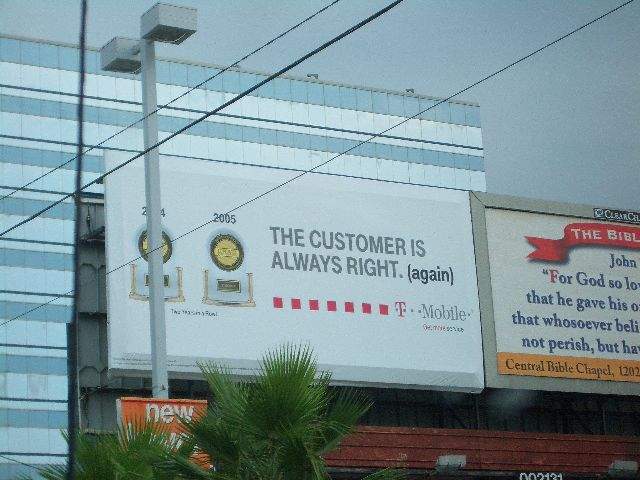This square-shaped, low-resolution image depicts an outdoor scene under a light blue sky. Three black electrical wires stretch diagonally from the left to the upper right corner of the frame. Two billboards are present: one prominently positioned in the center with a white background, and the other partially obscured on the right side of the image, only a portion of it visible. Despite the pixelation and lack of clarity, the scene clearly captures a moment in a typical urban or suburban setting, defined by these distinct elements.